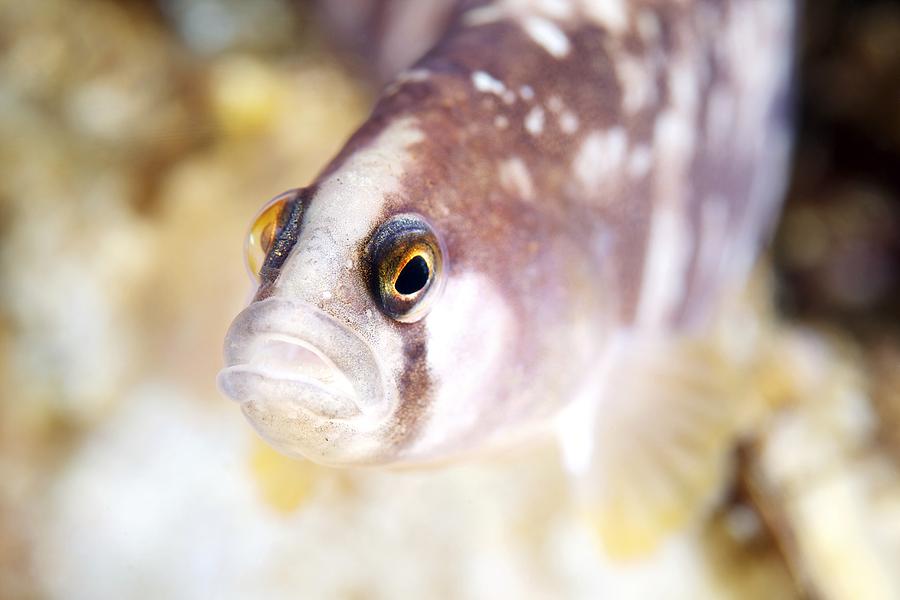This close-up photographic image captures the intriguing face of a tropical fish, prominently set amidst a blurry, aquatic background. The fish, resembling a goldfish, commands attention with its bulbous black eyes, surrounded by hints of gold and brown, giving an impression of them bulging outward. Its mouth is wide open, displaying thick, translucent lips with a hint of gray. The fish's head is predominantly white with a silver sheen between the eyes, transitioning into a purple-hued body adorned with brown and white spots. On the left side, a fin with a distinct yellow tip is visible, while the right fin has a translucent or gray appearance edged with yellow. The background, rendered out of focus, consists of shades of white, light brown, orange, and deep brown, which might be blurred rock formations or aquatic plants. Despite the image's graininess, the emphasis remains firmly on the fish's unique and expressive face.